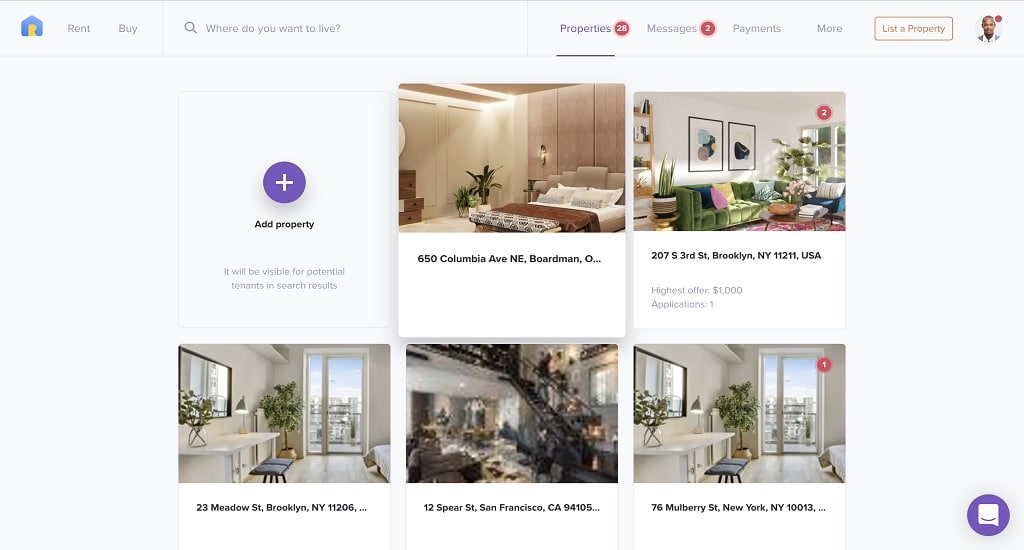The background is a solid gray color. In the upper left corner, there is an icon of a blue house with what appears to be a yellow or orange keyhole design. To the right of the house icon, the text "Rent or Buy" is displayed in gray, followed by a search bar with a magnifying glass icon. The placeholder text inside the search bar reads "Where do you want to live?" in gray. 

Below this, there is a navigation menu with options labeled "Properties" (showing 28 properties), "Messages," "Payments," and "More." Additionally, there is a profile picture of a Black gentleman looking straight ahead.

The main body of the page showcases five property listings. The first listing is empty and prompts the user to "Add a property," featuring a blue circle with a white checkmark and gray text underneath that says, "It will be visible for potential tenants to proceed."

The second listing displays a bedroom with the address "650 Columbia Avenue, Northeast Borman". 

The third listing shows a living room with white, sterile walls and is located at "207 East 3rd, Brooklyn".

The fourth listing features a very white and sterile room, located at "23 Metal Street, Brooklyn".

The fifth listing is of a two-story building with a black stairwell and predominantly white decor, although the photo is blurry. The address is "12 Spears Street, San Francisco".

The final listing presents another white, sterile room situated at "56 Murray Street, New York, New York".

The descriptions highlight the user's apparent preference for clean, white interiors.